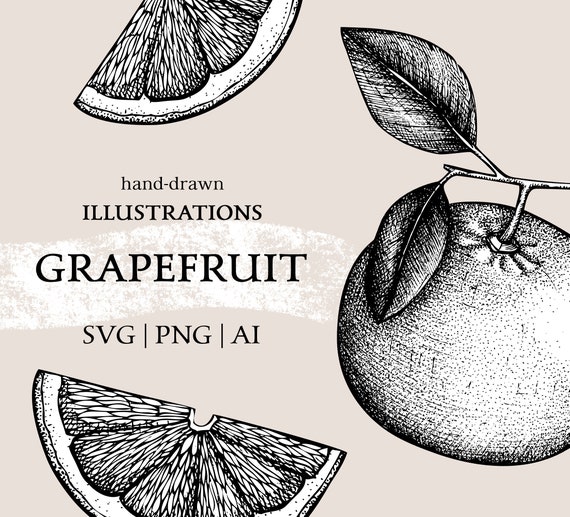This square image showcases a detailed, hand-drawn illustration of grapefruits against a pale background with a subtle strip of white across the center. In black pencil or charcoal, the artwork features a whole grapefruit with two leaves hanging from a limb on the right side. On the left, there are two slices of grapefruit - one at the top and one at the bottom, both slightly cut off. The illustration is labeled with large text that reads "Hand-drawn Illustrations" and "Grapefruit," followed by "SVG," "PNG," and "AI" separated by vertical lines. The background color varies slightly in description, ranging from light gray to a very light brown or soft violet, indicating nuanced tones in the image.